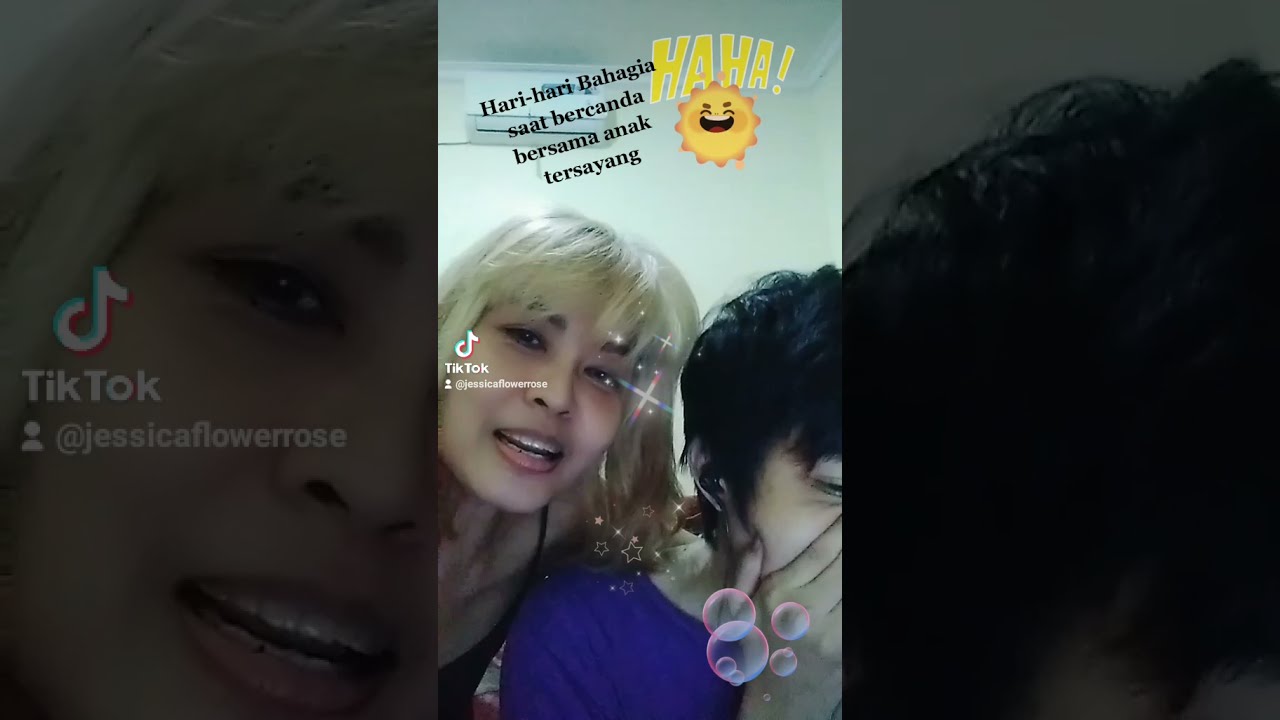The image is a rectangular, horizontally oriented screen grab from TikTok, featuring two young women. The background is slightly blurry compared to the clear foreground, emphasizing the close-ups and details. On the left and right sides, there are vertical, slightly transparent black bars. The bar on the left shows a close-up of the left woman's eye and blonde hair, and in this section, there is text that reads "TikTok" and "Jessica Flower Rose." The center of the image shows a color photo of two women, likely of Asian descent, laughing and having a good time in a white room. The woman on the left features bleach blonde hair with dark black eyebrows and bangs, while the woman on the right has short black hair and her hand cupped over her nose and mouth, possibly signaling laughter or surprise. The right vertical bar captures a close-up of the right woman's head, highlighting her black hair. Over the top of the central image are foreign-language words, and in bright yellow English text, it says "ha-ha!" with an animated smiling sun. The image also features graphics of stars and pink bubbles, adding a playful, cheerful atmosphere.